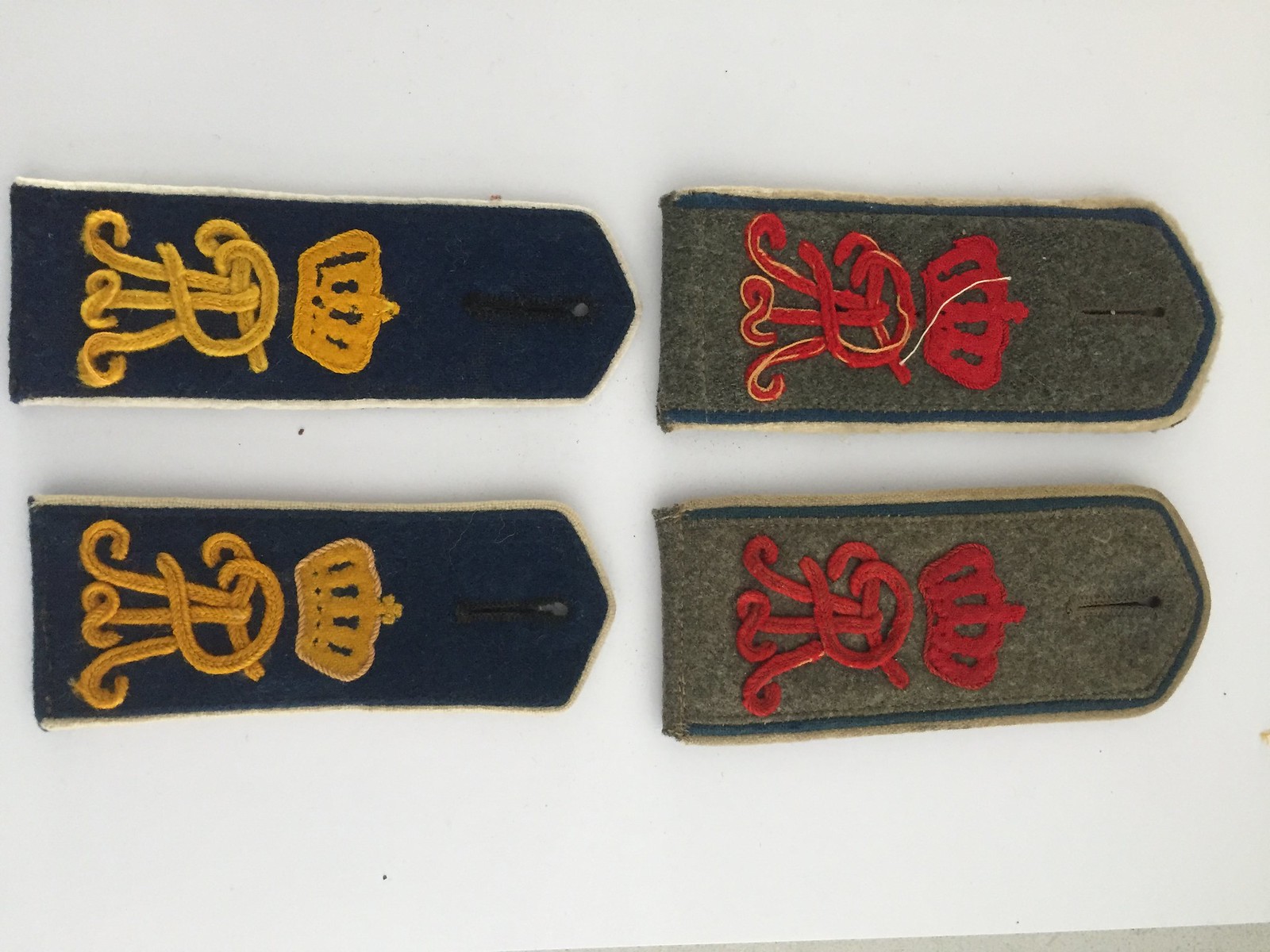This photograph features four military-style epaulets neatly arranged on a plain white background, all facing from left to right and stacked horizontally. Each epaulet is a long rectangle with a triangle tip at the bottom and a buttonhole near the top for attachment. The left two epaulets are a navy blue background adorned with a detailed gold-embroidered design. This design includes a thick, ornate crown on top, followed by an intricate, looping "R" beneath it. The right two epaulets have a darker gray background with similar blue and tan borders. They feature the same design, but in red embroidery with white and tan accents, including a detailed red crown and a fancy red "R" below it. Each epaulet showcases fine craftsmanship, blending military formality with decorative elegance.